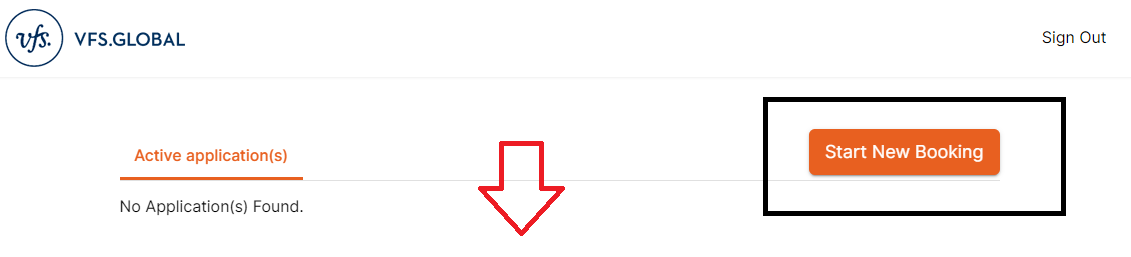Screenshot of the VFS Global website interface. 

The VFS Global logo is displayed prominently on the upper left corner of the screen. The logo features a lowercase "vfs" in blue, script-style text with a dot at the end, encapsulated in a thin blue circle. To the right of the logo, "VFS.GLOBAL" is shown in uppercase blue text. 

In the upper right corner, a "Sign Out" button is visible as plain text.

The main content area is structured into sections. At the top, in orange text, "Active Application(s)" is displayed, with a red underline beneath it. Directly below, in blue text, "No Application(s) Found" is noted. 

To the right of this text, there's an orange button with white text that reads "Start New Booking". 

This button is surrounded by a black rectangular highlight and a downward-facing arrow outlined in red, pointing towards the button, indicating interaction or emphasis on this area. 

The horizontal layout is further defined by a gray line that spans the width of this section, situated underneath the "Active Application(s)" text and aligning with the right side of the "Start New Booking" button.

The rest of the screen is predominantly white, providing a simple and clean user interface without additional elements.